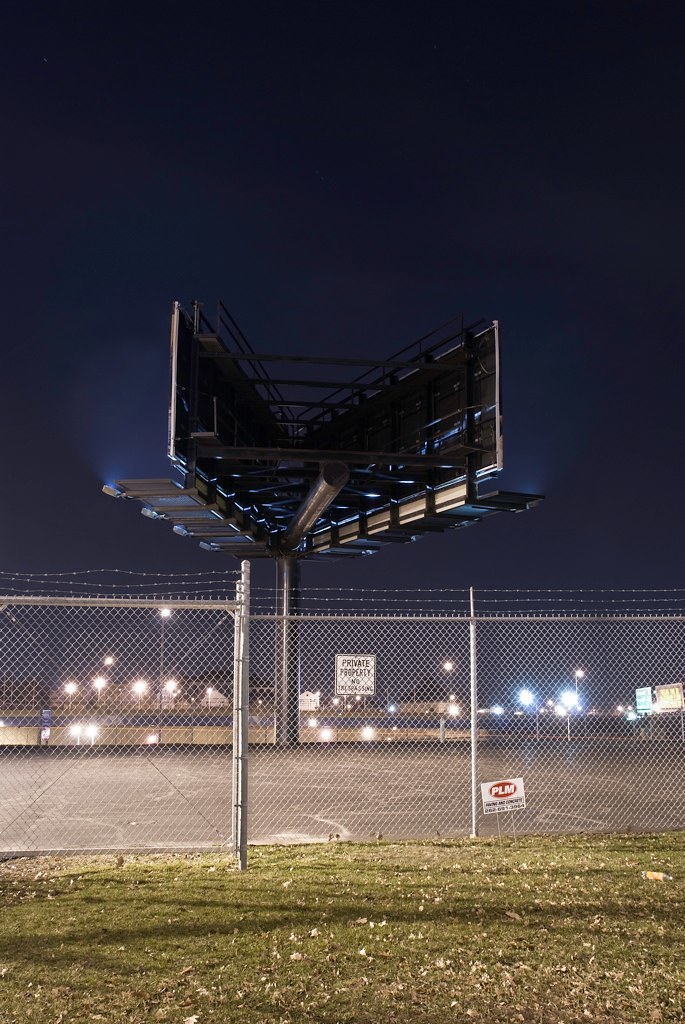In the nighttime photograph, the dark, slightly cloudy, blackish-blue sky looms overhead, devoid of any moon or stars. In the foreground, a well-manicured grassy area stretches out, accentuated by patches of beige foliage. A tall chain-link fence topped with several strands of barbed wire borders the grass. Attached to the fence are two white signs, one cautioning "private property" and another smaller, partially illegible sign marked with "PLM" and other text.

Behind the fence lies an urban parking lot, illuminated by a series of yellow and bluish streetlights. The scene also features two massive billboards mounted on a singular, sturdy black pole. These billboards are positioned back-to-back, facing opposite directions, with their skeletal metal support structure visible but their content unreadable from this vantage point. The distant backdrop includes additional illuminated white signs and several low buildings, indicating a bustling urban area.